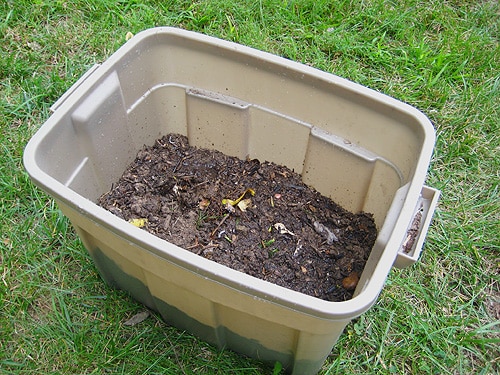The photograph in landscape layout captures a plastic tote, approximately 25% filled with a mixture of brown dirt, dead leaves, small branches, and possibly some mulch, situated on a lush, green lawn. The tote, which appears tan with a hint of gray, is positioned diagonally, extending from the top left to the bottom right of the image, with visible handles on both sides. The contents seem to be a collection of debris possibly cleaned out from gutters, ready for disposal. The grass around the tote is notably healthy and tall, creating a striking contrast against the more muted colors of the tote and its contents. No people or additional objects are present in the image, highlighting the simplicity of the scene.